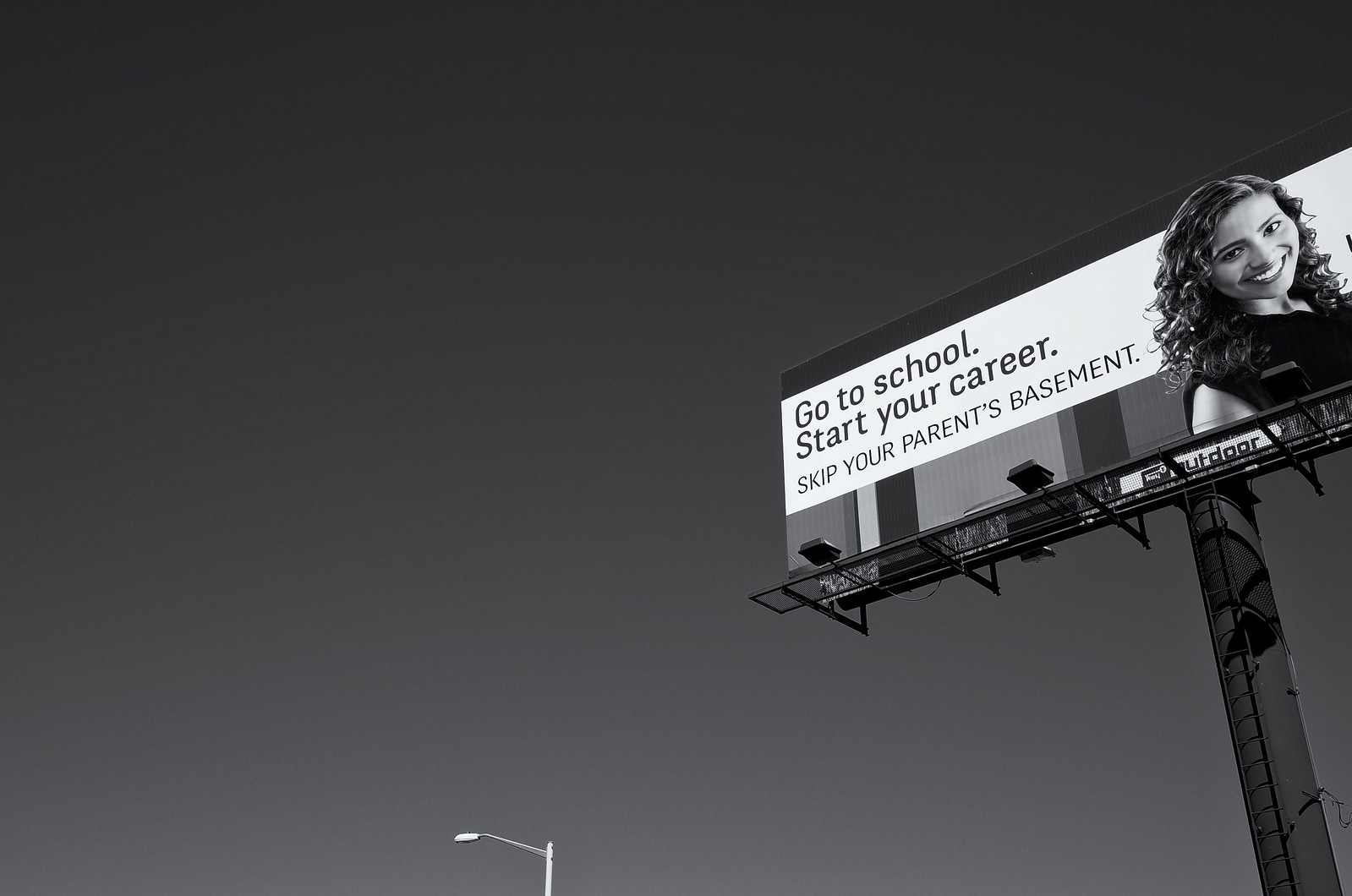In this captivating black and white photograph, the background transitions from a deep black at the top to a light gray at the bottom, creating a dramatic gradient effect. Prominently featured in the background is a white streetlight, which stands out against the darker surroundings. 

At the bottom center of the image, the top of the streetlight is clearly visible. On the right side, a black post is affixed to a towering billboard, which is accessed by a black ladder that ascends to the structure. Four supporting posts are seen protruding from the billboard.

The billboard itself is predominantly white with a compelling advertisement. On the right side of the billboard, there is an image of a woman with curly dark hair, beaming a bright smile. She is dressed in a black short-sleeve shirt. The text on the billboard reads: "Go to school, start your career, skip your parents' basement." This juxtaposition of the grayscale photograph with the encouraging message on the billboard adds a layer of nostalgia and motivation to the scene.